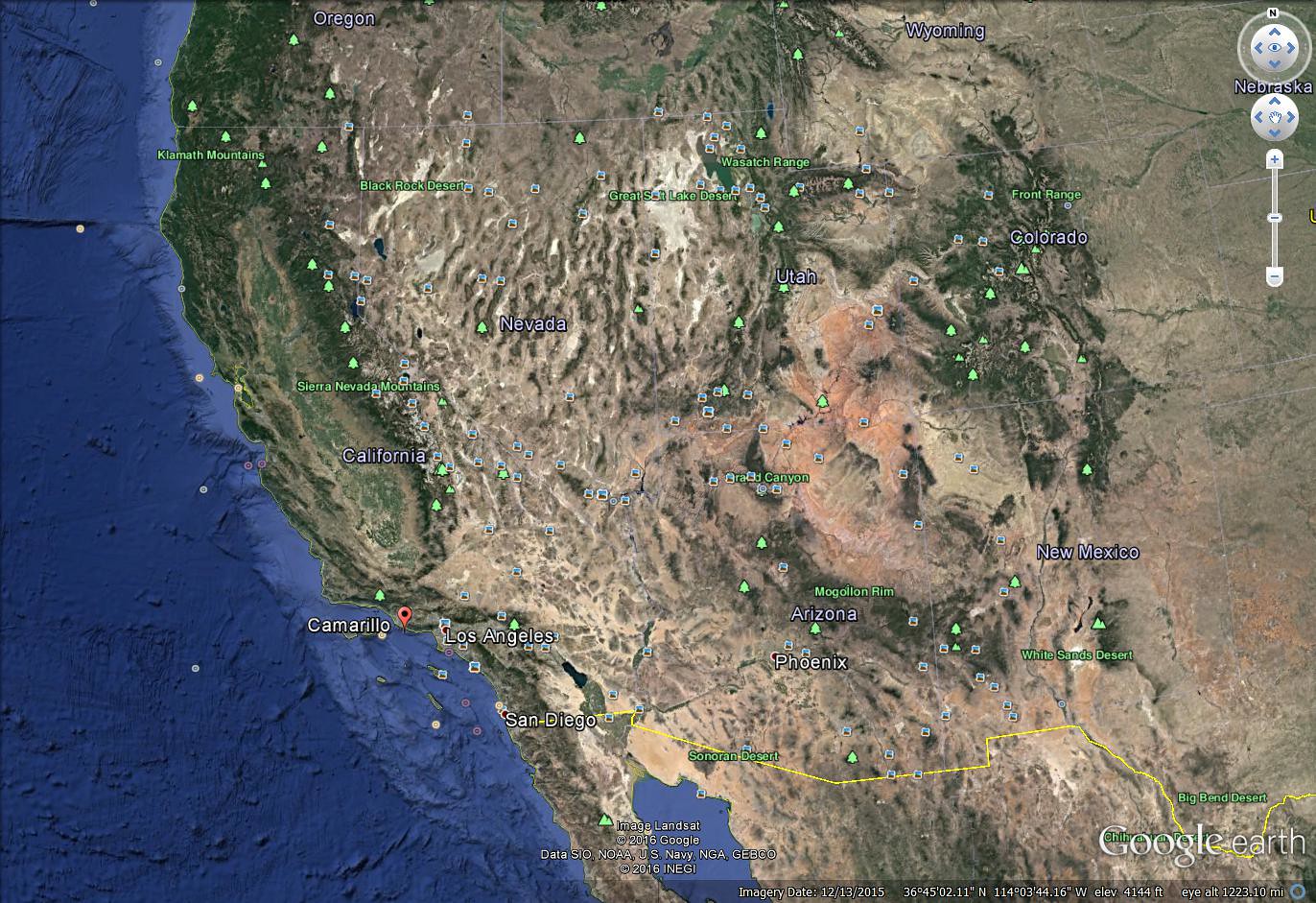The image displays a Google Earth map focusing on the western portion of the United States. Visible states include California, Nevada, Oregon, Washington, Idaho, Utah, Arizona, New Mexico, and parts of Colorado. Various geographical and urban points of interest are labeled, including major cities like Los Angeles and prominent mountain ranges. The map spans from the Pacific Ocean on the west to approximately halfway through Colorado and New Mexico on the east. The user interface elements are evident, with a navigational display in the upper right corner allowing for directional movement and zooming capabilities. The Google Earth watermark is situated in the bottom right corner, alongside a listing of image sources in the same area, providing the context for the displayed imagery.